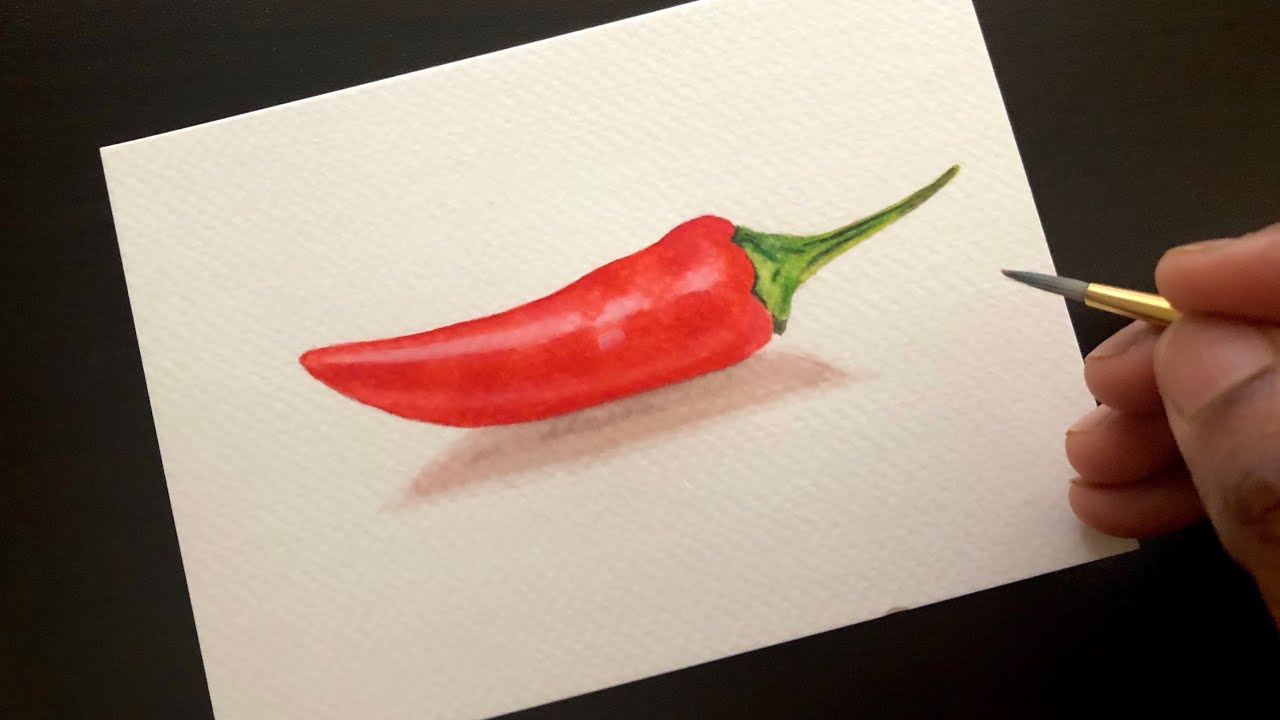The photograph, set against a black background, features a detailed watercolor illustration of a red chili pepper with a green stem, positioned diagonally across a white, textured watercolor paper. The paper is angled upwards to the right, where a left hand with darker brown skin tones is visible, holding a fine-tipped paintbrush with a gold ferrule. A subtle shadow beneath the chili pepper enhances its realistic appearance, though the shadow's rectangular shape contrasts with the pepper's form. The overall composition suggests a demonstration or an advertisement, likely intended for a digital art platform.